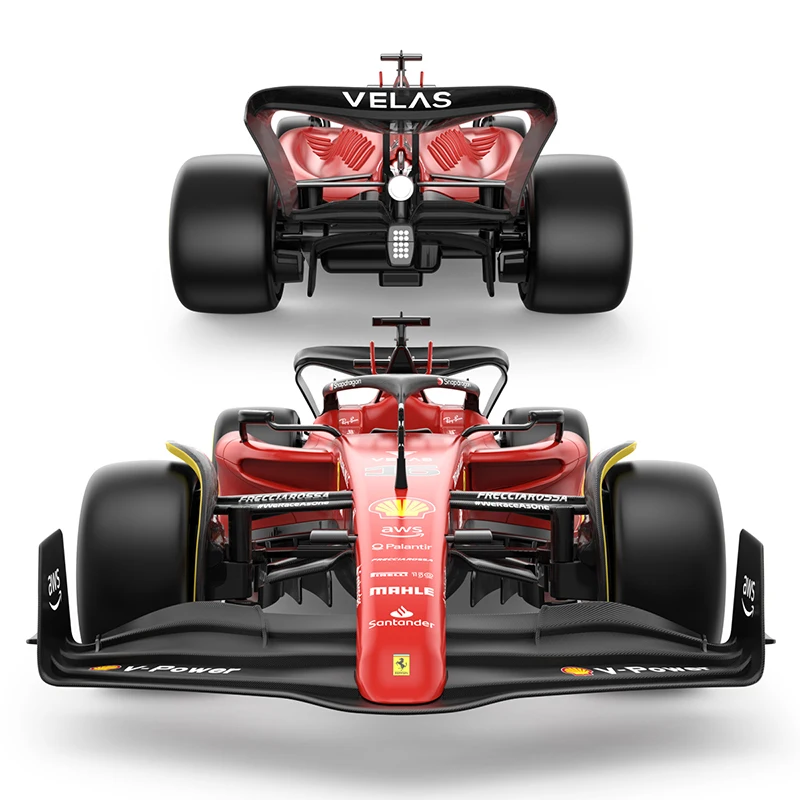The image shows a detailed view of a red Formula One race car, depicted in two parts: the top section displays the rear and the bottom section showcases the front. The race car has prominent black accents and treadless slick tires. On the back, "VELAS" is prominently displayed in white letters. The rear features a wind vane and a visible roll bar. The front displays various brand logos, including V-Power, Shell, and AWS. Notably, the front includes a black vane that runs side to side, designed to maintain ground contact. The image is well-lit against a white background, providing a clear and detailed view of the race car's features.